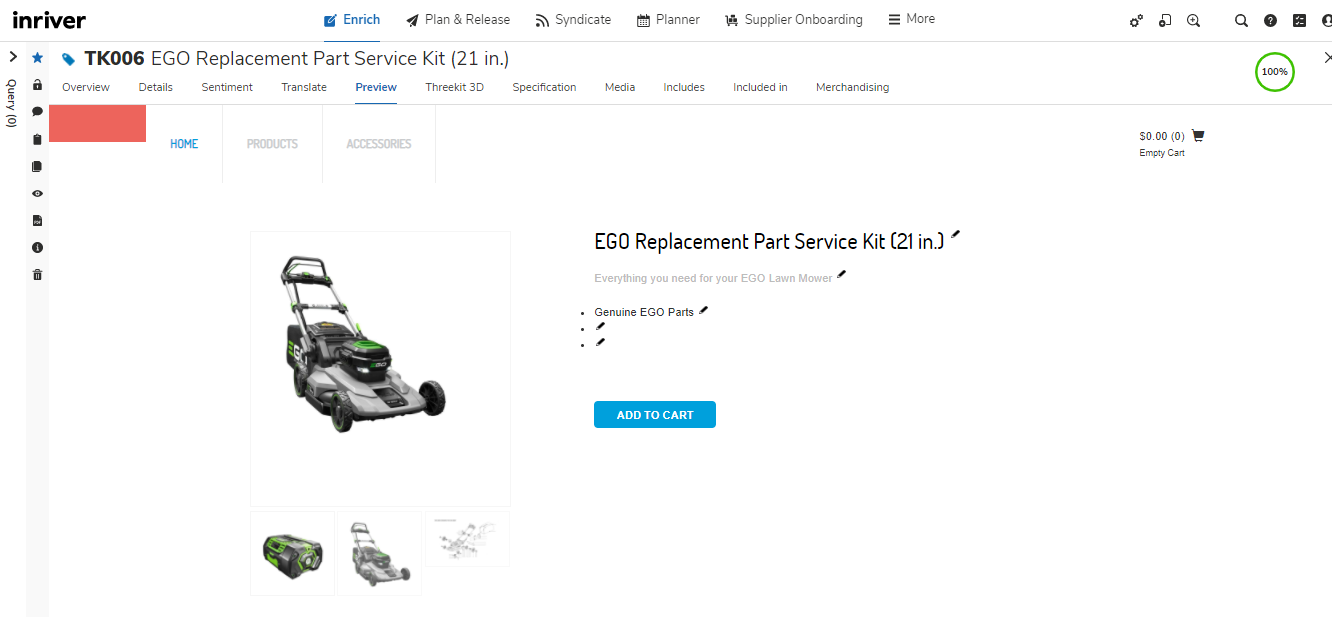This is a detailed description of a screenshot from the shopping website InRiver. The website features a white background. In the upper left-hand corner, "InRiver" is displayed in bold black letters, followed by "Enrich" in blue, indicating it's highlighted. Moving right, there is an upward-facing arrow, and next to it, in black letters, are the words "Plan and Release." Further to the right, a small black icon with two half-moon shapes over a dot is labeled "Syndicate," also in black. Next is a calendar icon labeled "Planner" in black. Further to the right, "Supplier Onboarding" is written next to a small, hard-to-see black icon. 

Farther right, there are three horizontal lines labeled "More." The extreme right side resembles a standard computer browser interface, complete with a zoom button, magnifying glass search icon, a gray circle with a white question mark inside, and a three-quarter gray box with a dark gray top right corner. Another small, partially cut-off image appears at the far right.

The main content below this menu features a blue ticket icon labeled "TK006" in bold black letters, followed by "EGO Replacement Part Service Kit, 21 inches." Beneath this are several tabs labeled "Overview," "Details," "Sentiment," "Translate," "Preview" (highlighted in blue), "Throw Kit 3D," and "Specification," followed by "Media," "Includes," "Included In," and "Merchandising." A green circle with "100%" in black is located at the far right of this section.

Further down, a red horizontal rectangle appears, to the right of which "Home" is highlighted in blue, followed by "Products" and "Accessories" in gray. Below this is an image of a gray lawnmower with green trim on the motor. To the right, the text reads "EGO Replacement Part Service Kit, 21 in." in black, followed by the description "Everything You Need for Your EGO Lawnmower" in gray. Below this description are bullet points stating "Genuine EGO Parts" with a pencil icon next to each. Further down, there's a blue "Descartes" button.

On the left side of this section are three thumbnail images. The leftmost appears to be a picture of the engine, the middle one depicts the entire lawnmower, and the rightmost shows the specific part in focus.